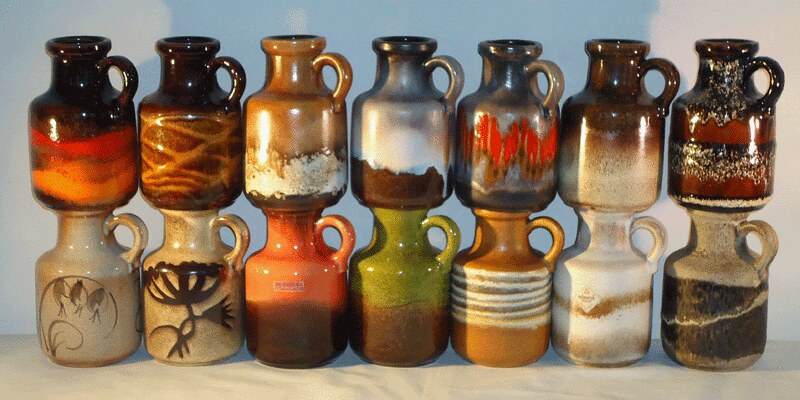This photograph showcases a collection of 16 handcrafted jugs meticulously arranged in two rows on a white marble countertop with gray accents. The setting appears dimly lit, and shadows of the jugs are cast on a white wall behind them. The jugs, each unique in design and color, feature predominantly dark tones such as browns, grays, oranges, and hints of blacks, reds, and whites. The handcrafted nature of the jugs is evident, with intricate patterns and swirls decorating their surfaces. The handles of these jugs are uniformly positioned towards the left, adding to the organized aesthetic of the display.